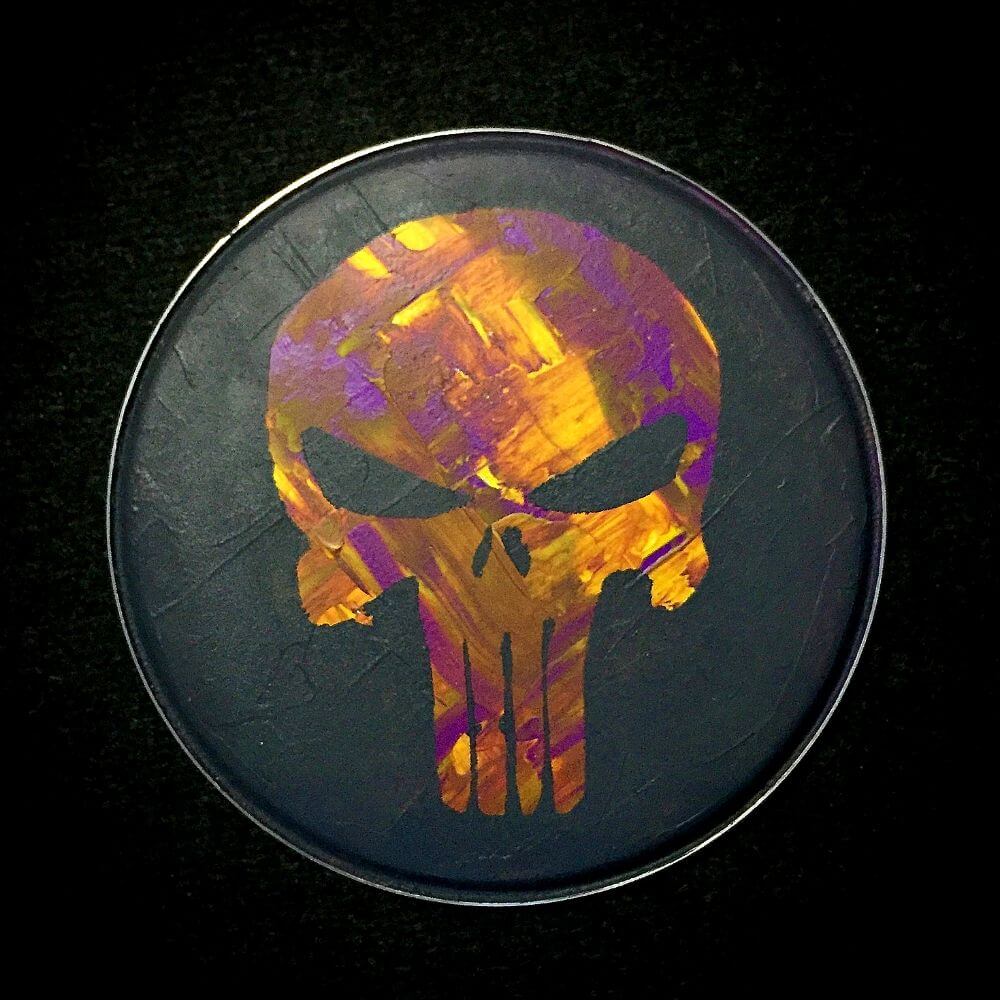The image features a captivating and textured depiction of the Punisher logo. Set against a plain, black background, the focal point of the image is a circular, button-like coin with a charcoal-gray hue and a detailed, rippled texture. The centerpiece of this coin is a painted version of the Punisher skull logo, rendered in striking hues of orange, yellow, and purple. The elongated and jawless skull has an abstract and somewhat creepy appearance, with meticulously applied paint that suggests a reflective quality. The colors, while distinct, subtly blend at the edges, enhancing the overall visual complexity of the piece. The background, possibly resembling woven carpeting, transitions from very black at the edges to slightly lighter towards the center, highlighting the intricately painted and physically textured coin, which dominates the majority of the image.